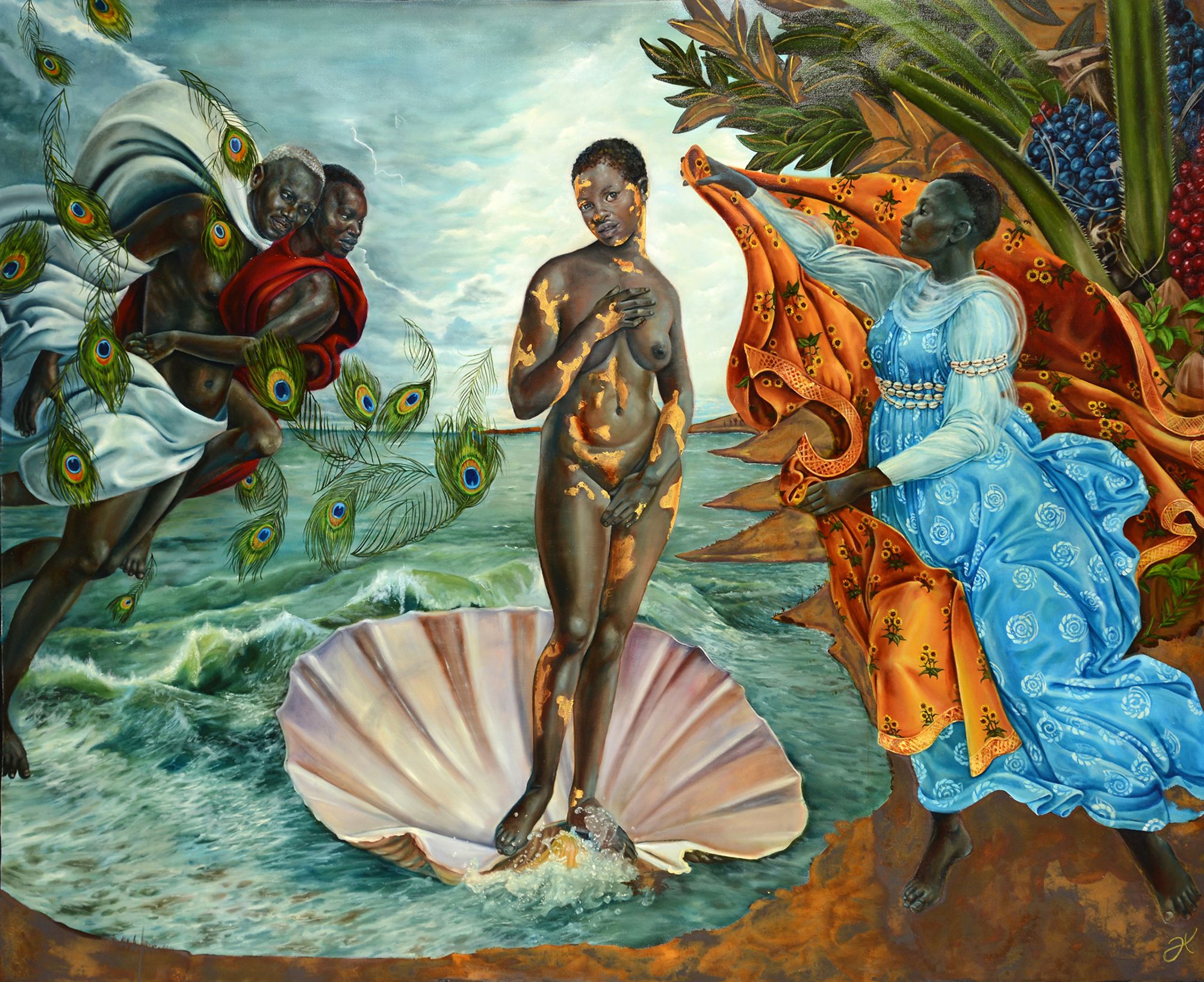The image is an illustrated color drawing with a detailed and vibrant scene reminiscent of Greek mythology. In the center, a dark-skinned woman with short, shaved hair stands gracefully in an open half-shell, echoing Botticelli's "The Birth of Venus." She is nude with gold blotches adorning her body, and while her left breast is exposed, her right arm is bent up, partially covering it. To her right is another black woman dressed in a flowing blue gown with lighter-colored sleeves and delicate white designs. She holds a large piece of orange fabric decorated with flowers, ready to cover the central figure. On the left side of the image, two black men are depicted; one carries the other on his back, both draped in white cloths. Surrounding them are peacock feathers cascading through the scene, adding to the ornate and mythical atmosphere. The background features rough ocean waters and a stormy sky lit with lightning bolts, enhancing the dramatic and dynamic composition. Behind the figures are plants with red and blue berries, contributing to the lush and vivid setting.